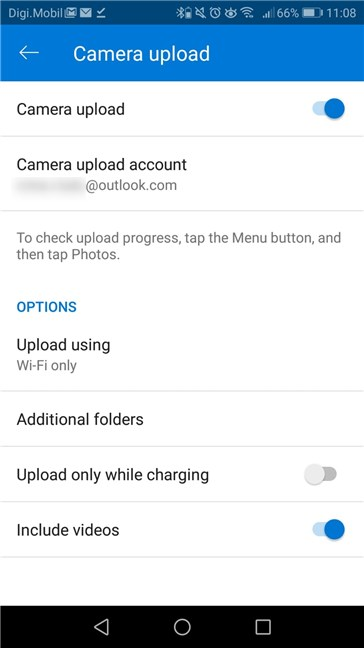This image is a detailed screenshot from a cell phone displaying the "Camera Upload" settings. At the very top, there is a blue rectangular bar spanning from left to right. On the left-hand side of this bar, there is a white, left-facing arrow. Centrally located on the bar, the text “Camera Upload” is written in white. 

Below the bar, on a white background, the text “Camera Upload” is prominently displayed in bold black letters on the top left, with a blue toggle button next to it indicating that this feature is turned on. 

Further down, aligning on the left, the text “Camera Upload Account” is shown in bold black letters, immediately followed by a blurred-out email address ending with "@outlook.com" in gray. 

Continuing down the image, there is a gray instructional text that reads, “To check upload progress, tap the menu button and then tap photos.” 

Below this instruction, on the left, the word “Options” is capitalized and highlighted in blue. Progressing downward, the text “Upload Using” appears in bold black letters followed by “Wi-Fi only” in gray beneath it. 

Further down on the left, “Additional Folders” is written in bold black letters, and under this, the phrase “Upload Only While Charging” is displayed in bold black letters. Adjacent to this phrase on the right side, there is a toggle switch that is turned off. 

Lastly, at the bottom left, the text “Include Videos” is shown in bold black letters, and to the right of this text, there is another toggle switch indicating that this option is turned on.